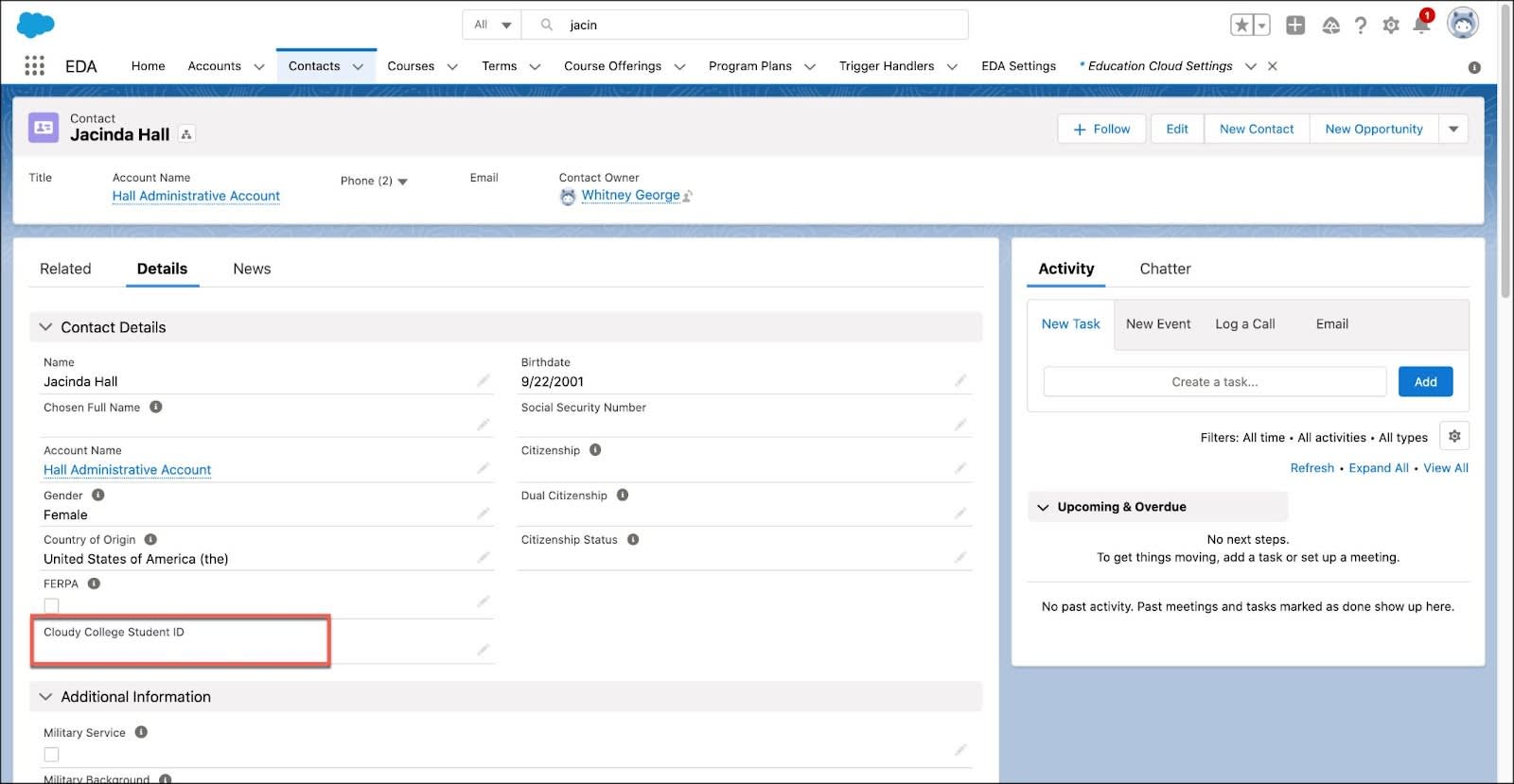This is an image of a computer interface created by a company named EDA, identifiable by their cloud and rain icon, which is predominantly blue. The central feature of this webpage is a contact profile for Jacinda Hall, with her name prominently displayed in large black letters. The top navigation bar includes options like "Home," "Accounts," "Contacts," and several other small, less readable tabs.

Below Jacinda Hall's name, there are various interactive buttons such as "Follow," "Edit," "New Contact," and "New Opportunity." The section beneath these buttons provides more detailed segments labeled "Related," "Details," "News," and "Contact Details." There is a red-outlined box indicating mandatory fields that require editing. This section includes fields for input such as name, account name, gender, country of origin, and birthdate, with several fields marked by asterisks to denote their necessity.

On the right side of the page, there are additional tabs labeled "Activity" and "Chatter," which likely provide further insights and communications related to the contact.